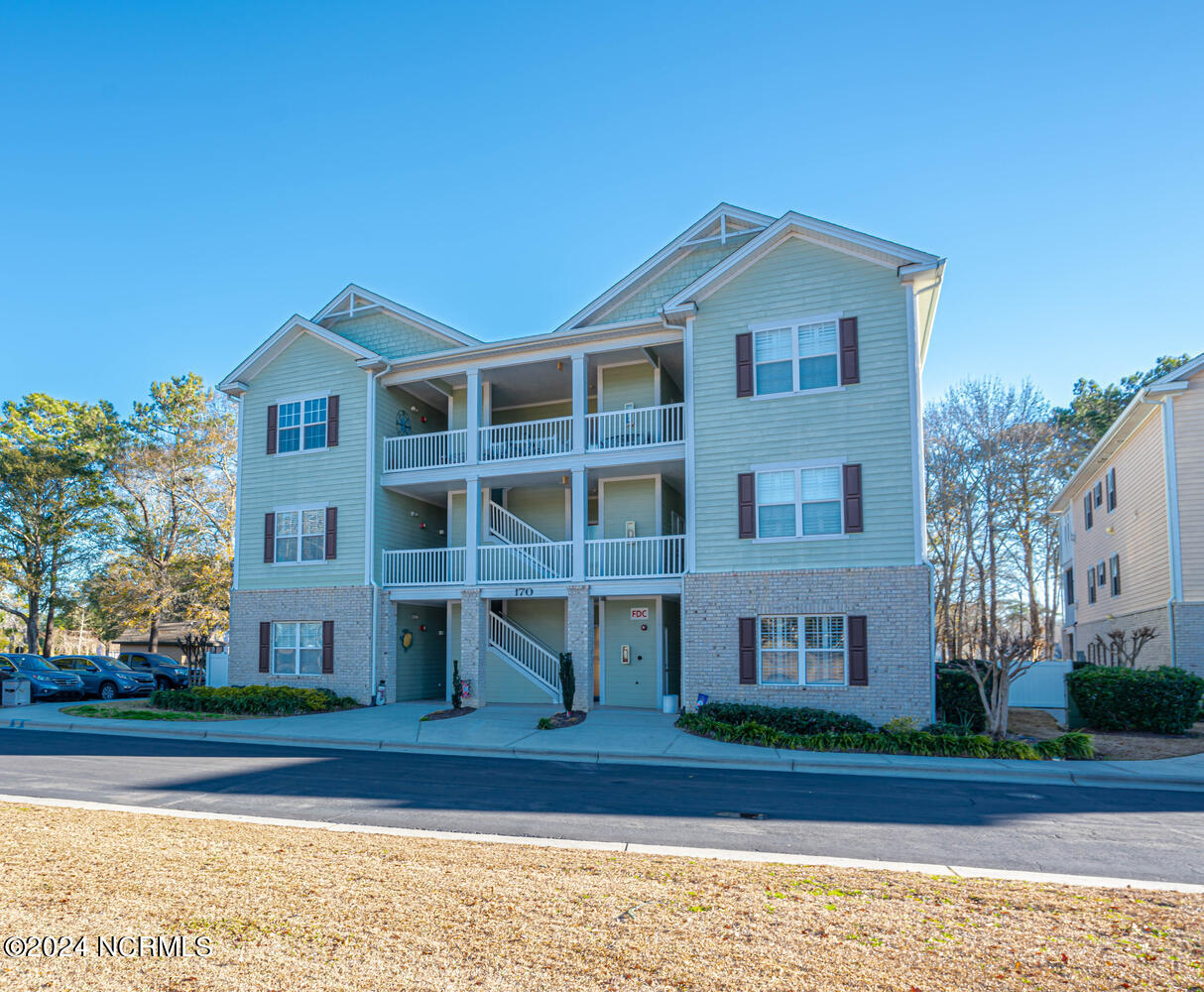The photorealistic image captures a three-story apartment complex standing behind a road, with dried brown grass in the foreground. The building's foundation is composed of a distinctive red brick, while the upper stories feature gray-greenish siding. Each floor has large double-sided windows with red panels, and there are prominent staircases and balcony landings on each level. 

To the right, a salmon-colored neighboring apartment building is visible, separated by a back alley and bordered by rows of bushes. In the left background, a parking lot with three cars, some likely Jeeps, and a pair of trees add more details to the scene. The sky transitions from deep blue on the left to lighter blue on the right. In the bottom left corner, a watermark reading 'Copyright 2024 NCRMIS' is present.